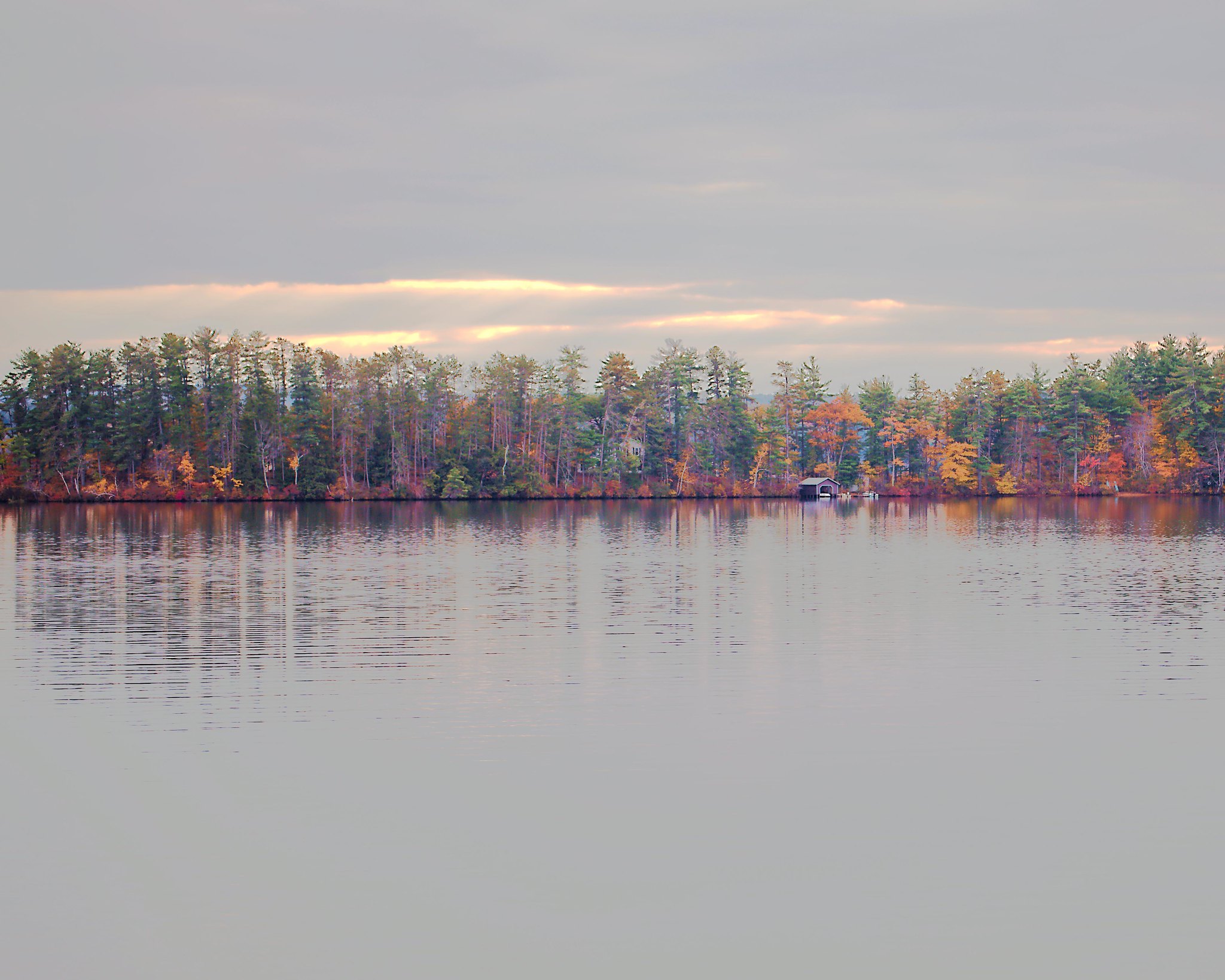A serene photograph captures a breathtaking lakeside autumn scene. The lake, occupying the bottom half of the frame, transitions from a matte gray at the forefront to a reflective surface closer to the vibrant forest, mirroring its vivid colors. The forest bursts with an array of fall hues, with lower sections ablaze in hot pinks, fiery reds, and warm oranges. Toward the right, the foliage transitions into brilliant yellows. Nestled amidst this colorful tapestry, a quaint purple house with a gray roof appears on the middle-right, its small size emphasizing the vastness of the natural surroundings. The sky above is heavily clouded, with the top part completely overcast. However, the lower section reveals gaps through which the sun pierces, casting a soft, golden glow across the scene, transitioning from orange on the peripheries to a radiant yellow towards the middle left. The treetops to the left edge of the image display a spectrum of greens and are distinctly individual due to the thinner forest density. On the right side, the trees are more densely packed, creating a lush blur of green pines.